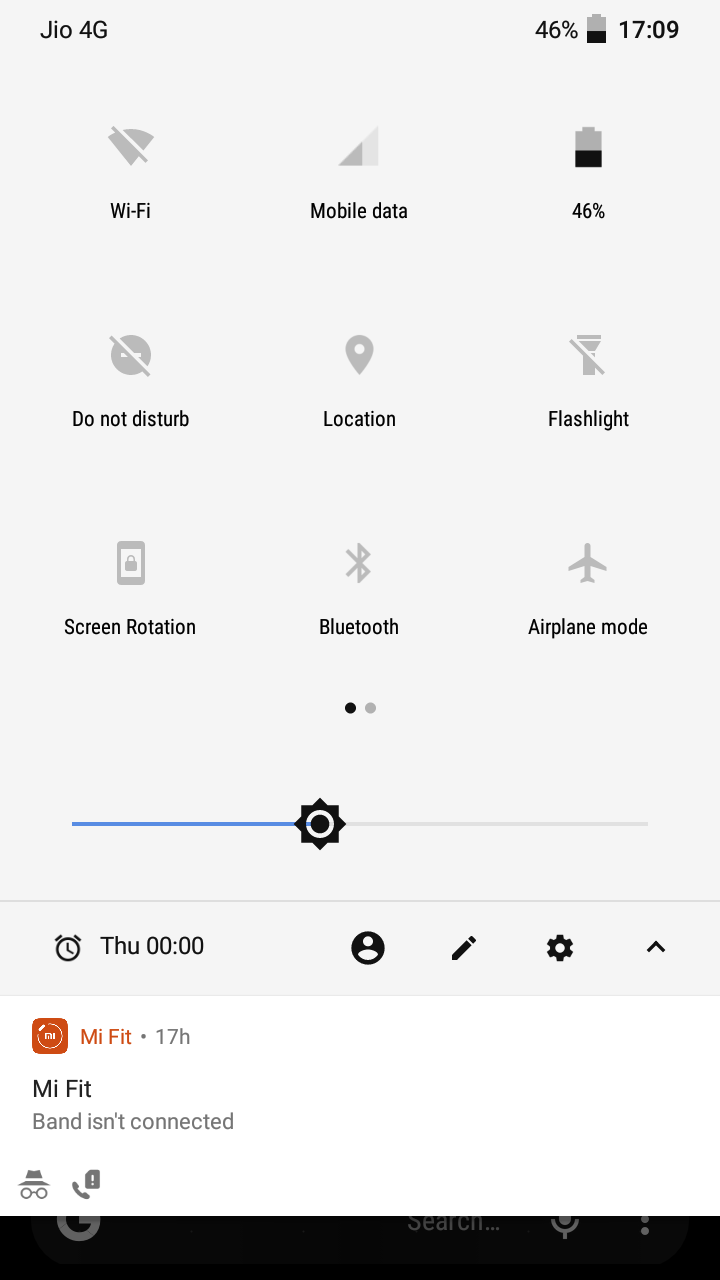A detailed caption for the image could be:

"The image shows a printed screenshot of a smartphone interface. At the top, the status bar indicates 'Geo 4G' as the network carrier with a 46% battery life at 17:09. Below the status bar, there are rows of icons representing various features: 'Wi-Fi,' 'Mobile Data,' (again showing 46% battery), 'Do Not Disturb,' 'Location,' 'Flashlight,' 'Screen Rotation,' 'Bluetooth,' and 'Airplane Mode.' Each feature is represented by its respective icon. 

A blue divider partially runs along the left side, separating this section from the next row. The following line displays a clock and the text 'Thursday 00:00,' with four additional icons aligned to the right side. 

At the very bottom left, there is an orange-red icon for the 'MI FIT' app, accompanied by the text '17 H' and a status message stating 'MI FIT band isn't connected.' Finally, the bottom of the image features icons for a hat, glasses, and a phone."